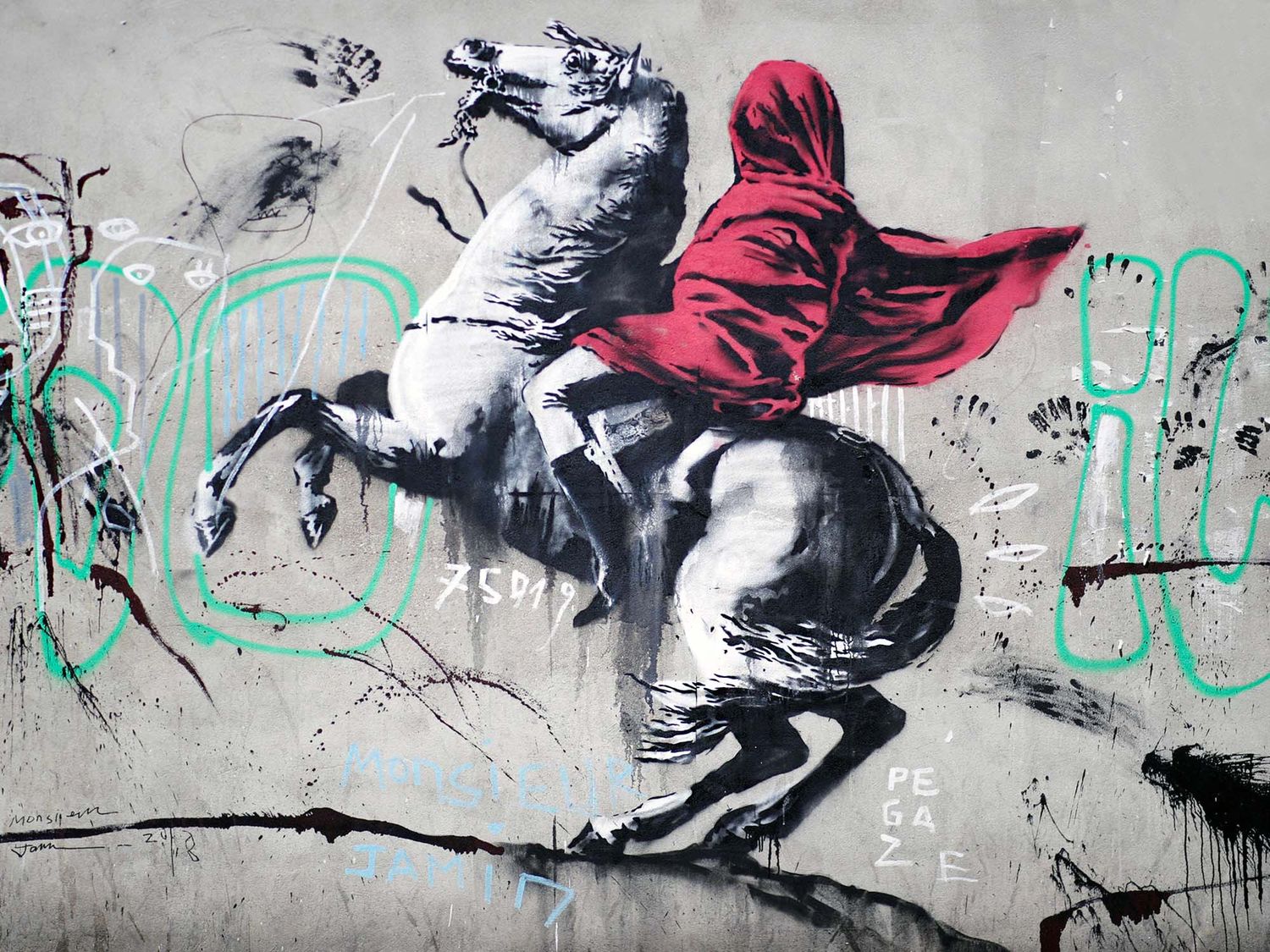The artwork is a detailed, square mural by the street artist Banksy, titled *Without Limits*. It features a reinterpretation of a famous painting of Napoleon on a white horse. The horse is rearing up on its hind legs with its mouth open, facing the top left corner of the image, and its tail towards the bottom right. Napoleon, the rider, is obscured from the legs upwards by a vivid red shroud that covers his entire upper body and head, leaving only his white pants and tall black boots visible.

The surrounding environment includes various graffiti elements on a light gray stone-like background without a definitive border. On the right side, there’s blue lettering that reads "I.U.", and in the lower right corner, there’s the word "P.E.G.A.Z.E." underneath the horse's hooves, along with the number "75D19". The left side features abstract graffiti including green outlines, black scribbles, faces drawn in a cubism style, white stick figures, and black ink splatters. This richly detailed mural, blending representational realism with street art elements, adds depth and intrigue to the classical imagery.